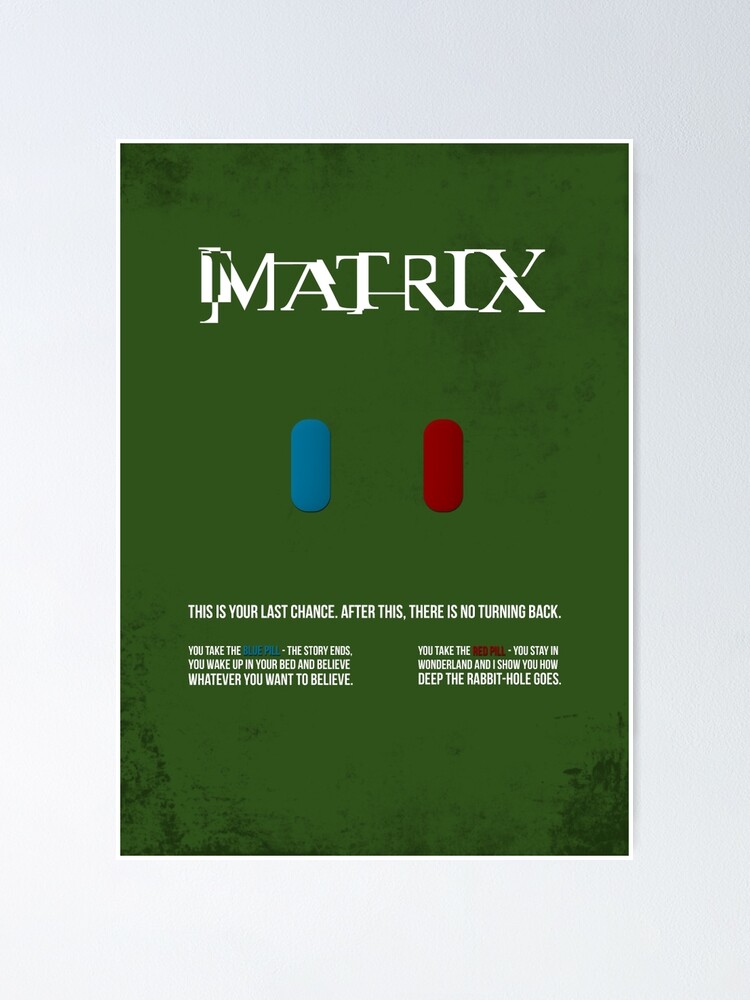A highly detailed digital rendering of a redesigned poster for the iconic film "The Matrix" adorns a white wall. At the top of the poster, in the distinctive Matrix font, the word "MATRIX" stands out against an olive-green, grungy background. Below the title, two capsules are prominently displayed: a medium blue pill and a dark red pill, representing the film's famous choice. Below these pills, the poster features a well-known quote from the movie in sans-serif font: "This is your last chance. After this, there is no turning back." Further detailed text reads, "You take the blue pill, the story ends, you wake up in your bed and believe whatever you want to believe. You take the red pill, you stay in Wonderland, and I show you how deep the rabbit hole goes." The text is in all caps and displayed in white, segmented appropriately with punctuation as described. The bottom of the poster becomes shadowy and darker green, adding to the visual depth and maintaining the dystopian aesthetic of the film.